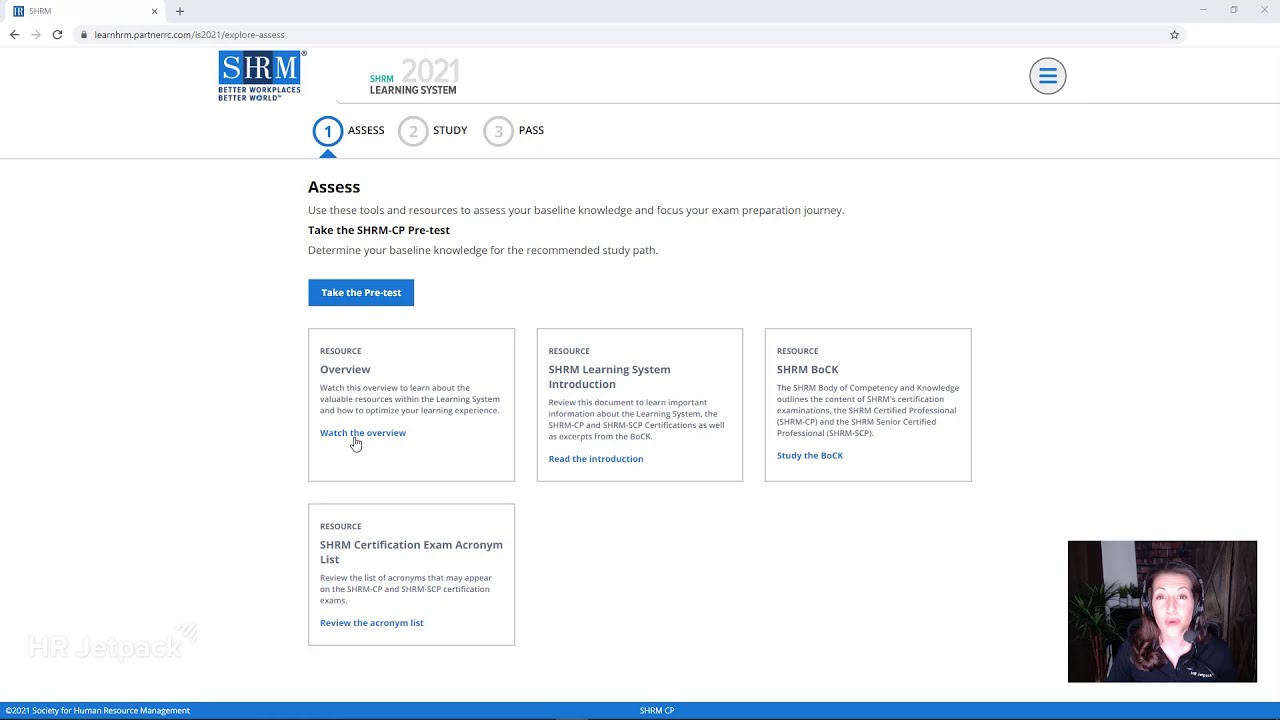Screenshot Description:

This image is a screenshot captured from a laptop displaying a webpage from the SHRM (Society for Human Resource Management) website. The browser window prominently features the SHRM logo, which is composed of the letters "S" and "M" in a bright blue background with white lettering, and "HR" against a navy blue background.

On the right side of the webpage, there are navigation tabs plainly visible. These tabs are sequentially numbered within blue circles: a "1" labeled "Assess," a "2" labeled "Study," and a "3" labeled "Pass."

Despite the small print making the rest of the text difficult to decipher, various blocks of textual content are scattered across the page. In the bottom right corner of the screenshot, there is a small image of a woman, potentially from a live webcam feed or a displayed profile picture. She appears to be wearing a navy blue top with a collar.